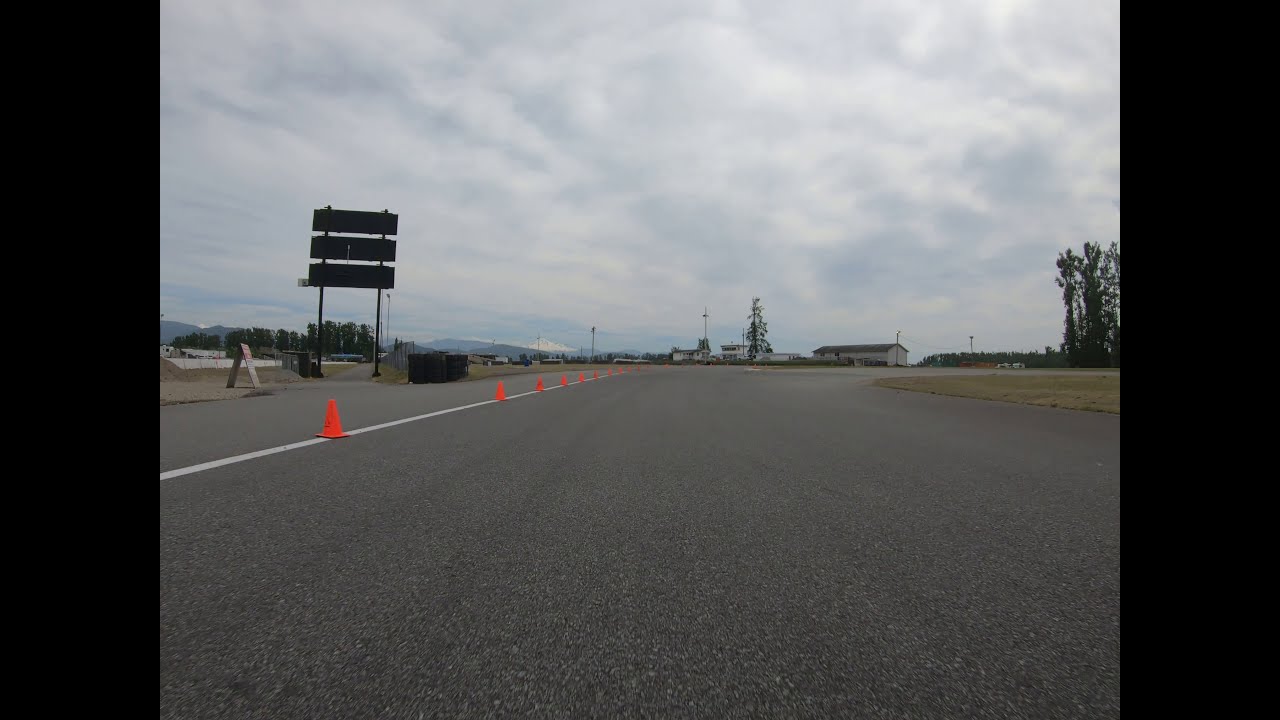The photograph showcases a vast expanse of asphalt, potentially an airstrip or roadway, under a cloudy, overcast sky. The prominent feature is a line of small, reddish-orange cones positioned along a painted white line that runs from the lower center-left of the image toward the center before fading into the distance. Adjacent to this line on the left side, there appears to be a border or pathway, possibly for pedestrians or cyclists. Further back on the left, a white stand with a black interior is visible. Behind this, a larger rectangular sign with three blank, black banners tops the scene. The background reveals a mix of single-story buildings and trees, with a tall tree and a row of trees lining the left and right sides of the image. In the extreme distance, mountains and light poles punctuate the horizon, adding depth to the otherwise stark landscape.